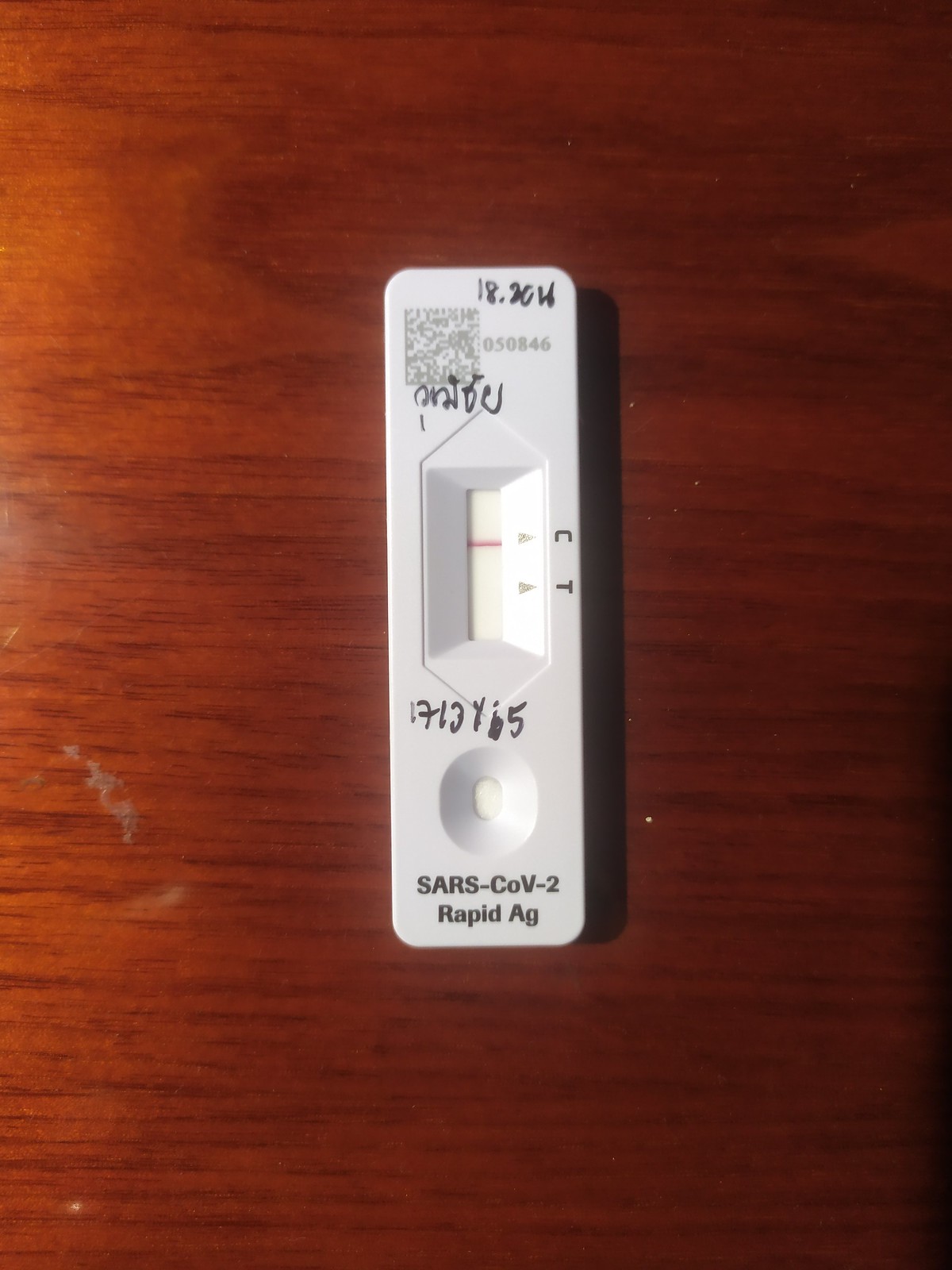This vertical color photograph depicts a SARS-CoV-2 rapid antigen test placed on a table. The test, made of white plastic, shows a single red line next to the letter "C" in its result window, indicating a negative result for COVID-19, with no line under the letter "T". At the top of the test, the handwritten notation "18.20h" is visible, accompanied by some illegible writing below it. Further down, another handwritten string reads "1713YI5". Additionally, the test features a serial number and a QR code, with the number "050846" positioned beside it. The table is bare, with the COVID-19 test being the focal point of the image.